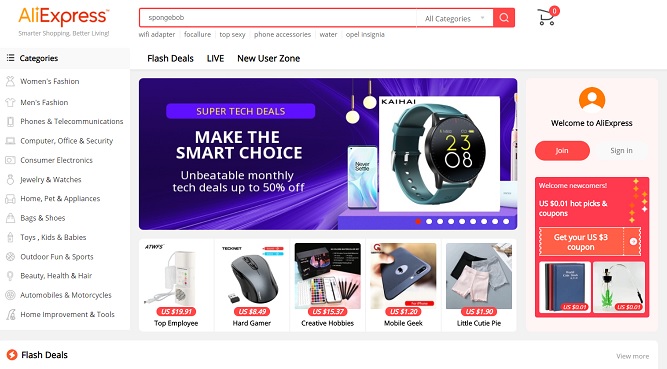The image depicts the homepage of an online store, specifically AliExpress. The AliExpress logo is prominently displayed at the top left corner, with "Ali" in yellow and "Express" in orange. To the right of the logo is a search bar with the term "Spongebob" entered. This search bar is outlined in orange, including the search button. The shopping cart icon, also orange, shows zero items. The background is predominantly white.

Below the AliExpress logo is the tagline "smarter shopping, better living." Adjacent to this on the right are various category tabs, including "wifi adapter," "focal," "top sexy phone accessories," "water," and "opening signal." Further tabs in black text like "Flash Deals" and "Live New User Zone" are also visible.

On the left side of the page, there is an extensive list of categories: women’s fashion, men’s fashion, phones and telecommunication, computer, office and security, consumer electronics, jewelry and watches, home, pets, appliances, bags and shoes, toys, kids and babies, outdoor fun and sport, beauty, health and hair, automobiles and motorcycles, and home improvement and tools.

The bottom section features the "Flash Deals" tab, below which is a highlighted product section. A specific device is advertised against a blue background, showcasing a promotion titled "Super Tech Deals" with the caption "make the smart choice, unbeatable monthly tech up to 50% off." To the right are images of a smartphone and a Kaihai smart watch, the latter displaying the time as 23:08 and featuring a green band against a black background.

Among the listed products are a "Toy Employee" priced at $19.91, a "Head Gamer Mouse" at $8.49, "Creative Hobby Makeup" for $15.37, a "Mobile Geek" smartphone cover for $1.20, and "Little Cutie Pie Shorts for Babies" priced at $1.90, with all prices marked in red.

On the right side of the page, it says "Welcome to AliExpress," including two buttons for user options—orange "Join" and "Sign In." Below this section is a welcoming message for newcomers, offering "$0.01 hotpicks and coupons" and a "$3 coupon" for US users.